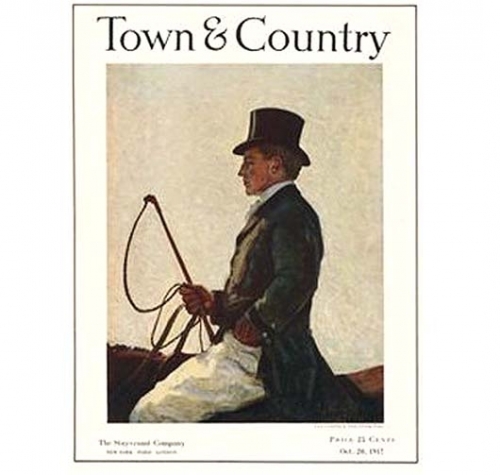This is the cover of a magazine called "Town and Country," set within a white frame with a very thin black border. At the top of the frame, the title "Town and Country" is prominently displayed in black letters. The central image features an English gentleman from the 1800s, characterized by his top hat, long black frock coat that fans out, and white trousers. He is seated on a horse, although only the top part of the horse is visible. The gentleman's right hand holds both the reins and a riding crop, while his left hand is casually placed in his pocket. A plain gray background serves as a backdrop, emphasizing the subject. At the bottom of the cover, there is blurred and faint text, with discernible words such as "Maryland company," and a partially legible date that appears to be either October 29th, 1917, or October 29th, 1967.